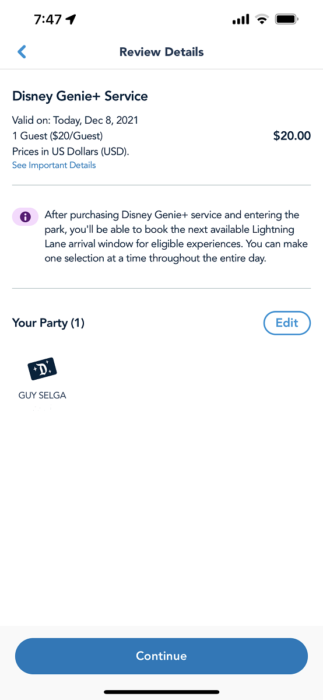**Caption:**

This screenshot captures a mobile phone screen displaying information about Disney's Genie+ service. The screen has a clean, white background with standard status indicators at the top. On the top-left, '7:47 AM' is displayed, followed by an arrow pointing northeast, indicating GPS activity. Adjacent to this, the phone shows full signal bars but lacks a visible Wi-Fi symbol. The battery icon beside it appears nearly full.

Beneath this status bar, centered on the screen, is a header that reads "Review Details," along with a blue back button on the top-left corner. The main content starts with a bold title: "Disney Genie+ Service," with the date in lighter gray below: "Valid on Today, December 8, 2021."

A breakdown of the service for "One guest" is listed next, noting the cost as "$20 per guest." This is reiterated on the right in darker gray as "$20." The following line states, "Prices in US Dollars," with "(USD)" in lighter gray.

Below this, a blue button labeled "See Important Details" is provided. The accompanying text explains the benefits of the Genie+ service: "After purchasing this and entering the park, you'll be able to book the next available Lightning Lane arrival window for eligible experiences. You can make one selection at a time throughout the access day."

Finally, it mentions that visitors can manage their party size and proceed by tapping the blue "Continue" button, designed to streamline one's experience at Disney World.